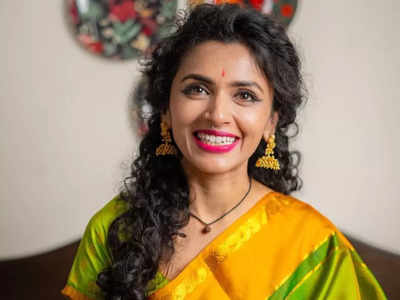This is a photograph of a woman, likely of Indian descent, sitting on a brown wooden bench. The backdrop features a white wall adorned with a partially visible, blurred art piece in a floral pattern. The woman has long, curly hair that cascades past her shoulders, teetering between black and dark brown. She is smiling warmly at the camera, wearing light purple lipstick and a prominent red bindi on her forehead, hinting at a cultural significance, possibly denoting marriage.

Her attire includes a traditional Indian dress, predominantly green with accents of yellow and possibly a touch of gold. An elegant yellow sash drapes over her shoulder. She accessorizes with decently sized gold earrings styled like brooches and a distinctive necklace with a black or brown rope, featuring a small brown stone pendant.

Her eyes are accentuated with black eyeliner, adding to her vibrant and joyful appearance. The entire composition captures her poised and graceful demeanor in a serene indoor setting.